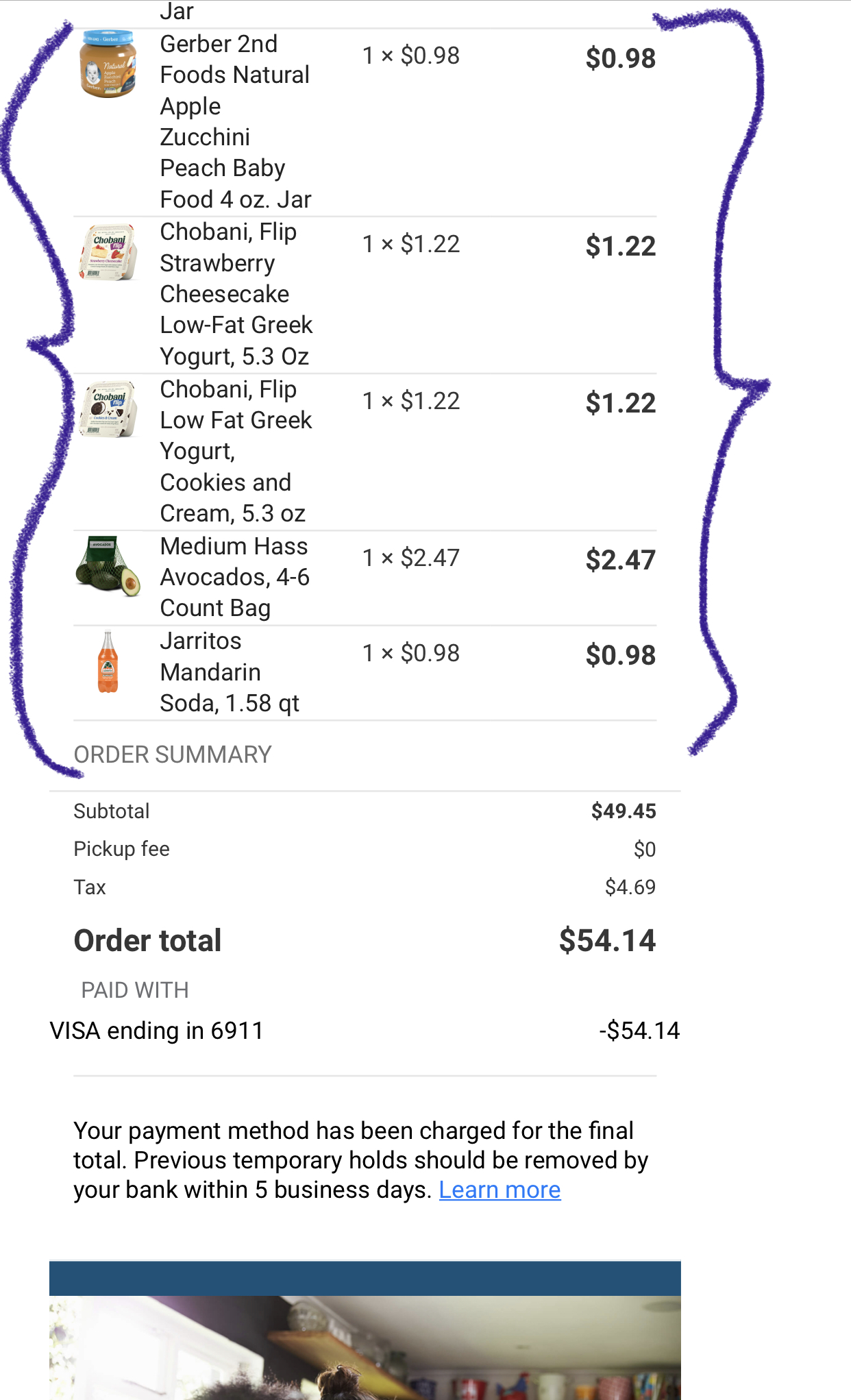A detailed screenshot of a mobile food order reveals various purchased items arranged in a summarized list. Starting from the top, each entry features a thumbnail image of the item on the left, followed by the item’s name, number of units, individual cost, and subtotal on the right. The items purchased include:

1. Gerber Foods Natural Apple, Zucchini, Peach Baby Food
2. Chobani Strawberry Cheesecake Yogurt
3. Chobani Cookies and Cream Yogurt
4. Avocados
5. Jermitos Mandarin Soda

Beneath the list, the subtotal for all items is provided, alongside applicable taxes, culminating in an order total of $54.14. The payment method is confirmed with a Visa card ending in 6911. The interface, indicating a mobile application, suggests that the order was placed using a smartphone, though the specific app remains unidentified.